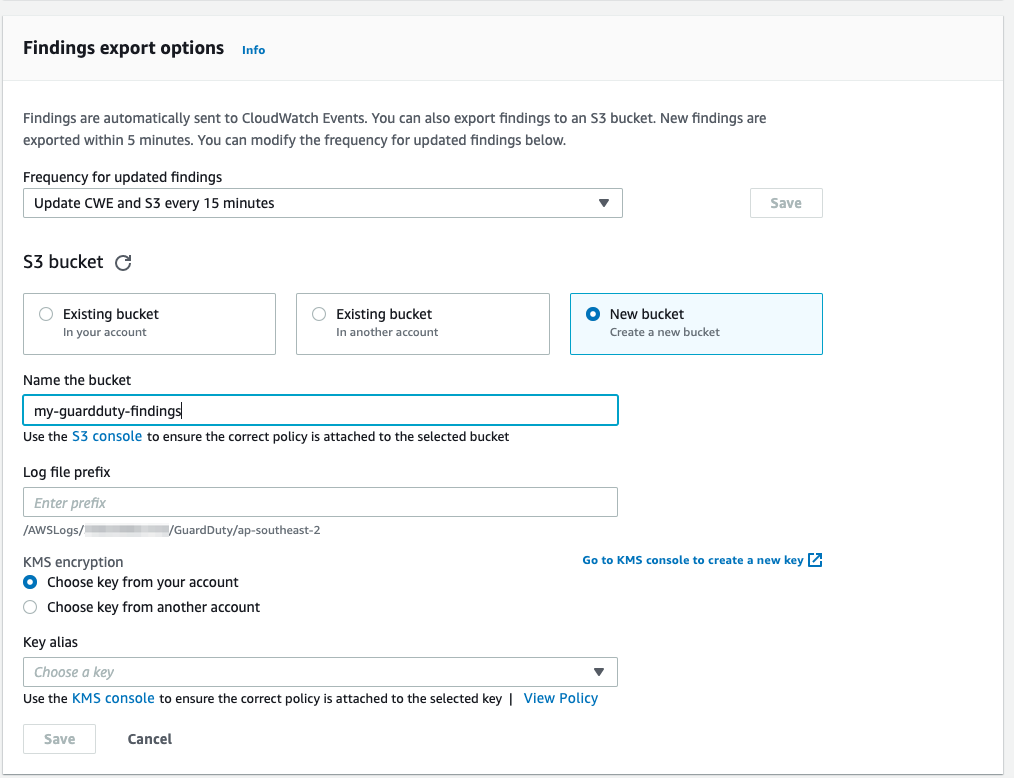The image appears to be a detailed interface for configuring export options in a software application. 

At the top, there's a segmented header with a lighter gray rectangle containing the text "Finding export options" in black and "Info" in blue. Below this, a description in black text reads: "Findings are automatically sent to CloudWatch Events. You can also export findings to an S3 bucket. New findings are exported within five minutes. You can modify the frequency for updating findings below."

The main body features several interactive elements:

1. A gray-outlined rectangular dropdown menu labeled "Frequency for updating findings" with the default selection "Update CWE and S3 every 15 minutes." An arrow on the right side allows for further adjustments.
   
2. To the right, another gray-outlined rectangle labeled "Save" in gray.

3. Below, there is a section with a header "S3 bucket," featuring:
   - A gray-outlined rectangle labeled "Existing bucket" with accompanying descriptive text.
   - Below this, another gray-outlined rectangle labeled "Existing bucket" with additional descriptive text.
   - Further down, a blue-outlined rectangle with a circle inside, labeled "New bucket" with more explanatory text.

4. Another section contains a label "Name of bucket" in black followed by a blue-outlined input field. Below this is a prompt "Use the S3 console" where "S3 console" is highlighted in blue, accompanied by guidance in black text: "to ensure the correct policy is attached to the selected bucket."

5. The next part of the interface includes a label "Log file prefix" followed by a gray-outlined input field, with some partially smudged text below it.

6. For KMS Encryption, there are options for selecting a key:
   - A blue-dotted circle option labeled "Choose key from your account."
   - A gray-outlined circle option labeled "Choose key from another account."

7. On the far right, some text is too small to decipher, but there is a gray-outlined rectangle with an upward-pointing arrow in the upper-left corner, labeled "Key Alias." 

8. Another input option labeled "Choose a key" with a downward-pointing arrow and text below that is mostly in black, although some words are in blue.

9. At the bottom of the interface, two buttons are present: one gray-outlined rectangle labeled "Save" in gray, and next to it, a black "Cancel" button. 

The interface is highly detailed and designed to give users control over how findings are exported and managed within an S3 bucket environment, with ample options for customization and security settings.